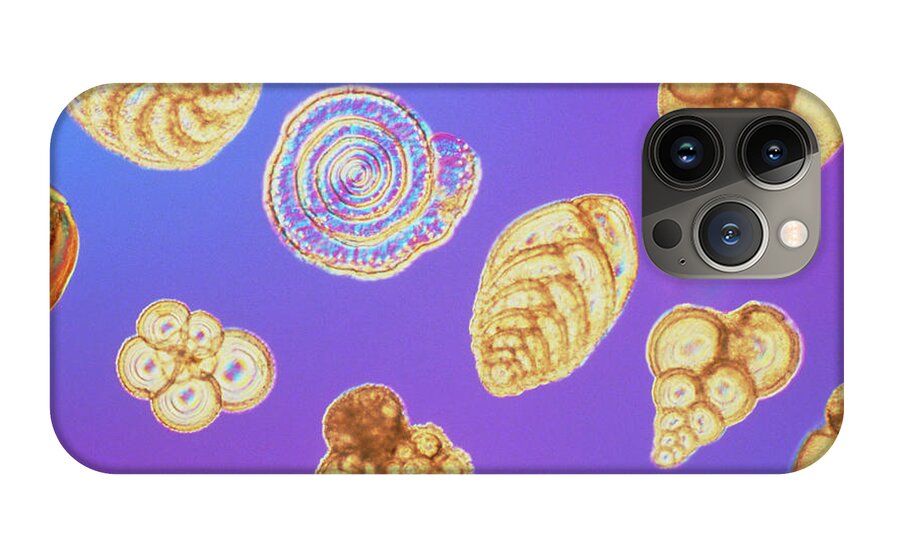The image features an iPhone, likely a newer model such as the iPhone 14, positioned horizontally. The phone itself is gray but is encased in a uniquely designed protective case. This case boasts a captivating gradient background, transitioning from a bluish-purple to a traditional purple hue. Overlaid on this vibrant background are various translucent yellowish, almost bubble-like designs that have a gentle rainbow sheen akin to soap bubbles. These designs include seven distinct cell-like groupings reminiscent of microscopic views, with shapes such as spiraling forms resembling snail shells and clusters of circles that vary in size. The case’s decorative elements also have shades of brown to light brown, adding a fossil-like or trilobite appearance. The three camera lenses and the flash of the iPhone are visible in the upper right section of the phone, indicating the case's precise fit and modern design.